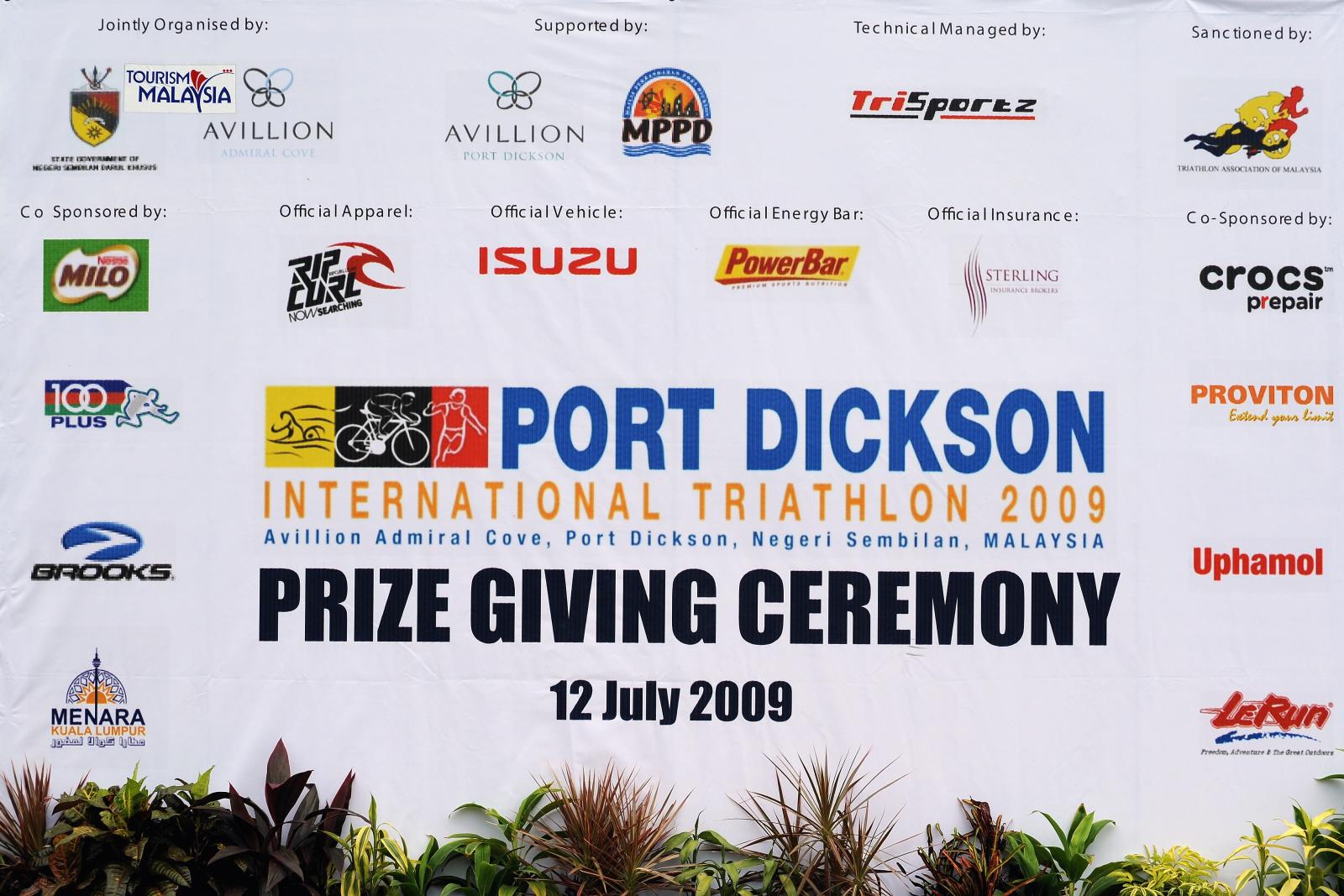The image depicts an event backdrop with a pale blue-gray background, filled with colorful icons and text. It prominently advertises the Port Dixon International Triathlon of 2009 held at Avillion Admiral Cove, Port Dixon, Negeri Sembilan, Malaysia. The text highlights the Prize Giving Ceremony which took place on 12th July 2009. Central to the design are symbols of the triathlon events: a swimmer on a yellow background, a cyclist on a black background, and a runner on a red background, accompanied by the event and location details in gold and black text. Surrounding the main text are various sponsor logos, including Tri Sports, Crocs, Proviton, Minara, Brooks, 100 Plus, Milo, Rip Curl, Isuzu, and Power Bar. The bottom part of the backdrop features a mix of green and brown plants, possibly artificial, adding a decorative touch.